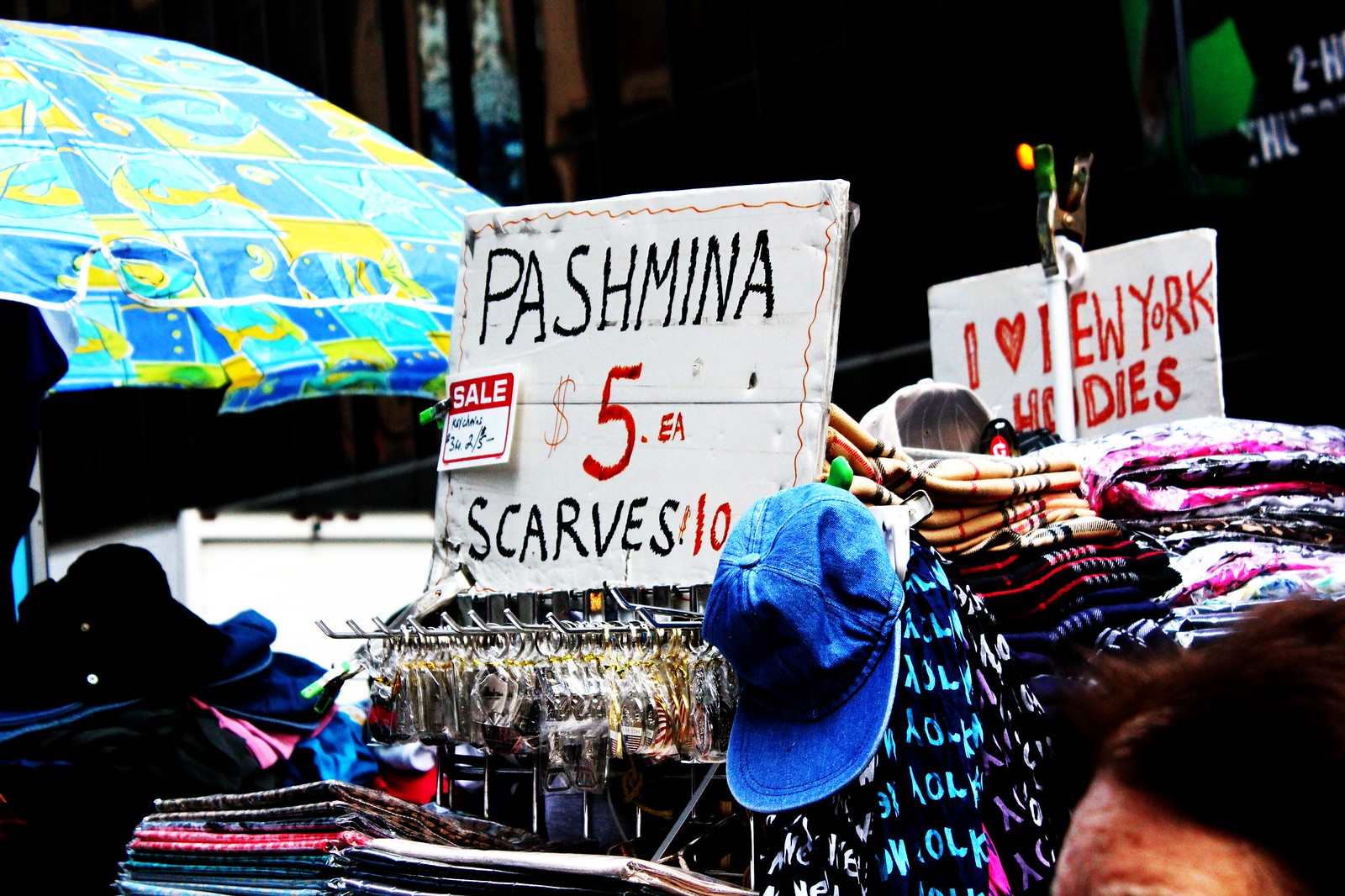The image captures a bustling outdoor market scene, likely in New York City, showcasing a variety of items for sale. On the left, there's a partially visible, vibrant umbrella with blue and yellow segments, hinting at a bodega setting. At the center stands a prominent, white sign in blue marker reading “Pashmina $5 each” and “Scarves $10 each,” with a smaller "sale" note on one side. Beneath the sign, and on the rotating rack it hangs from, are neatly folded pashminas, scarves, and a few key rings. To the right, another sign advertises "I Love New York" hoodies, accompanied by a pile of variously colored folded cloths, possibly T-shirts or beach towels also adorned with "I Love New York" prints. A single cap can be seen hanging, and just peeking into the frame at the bottom right is the partial view of a person's forehead and hair, adding a touch of human presence to the vibrant street market ambiance.